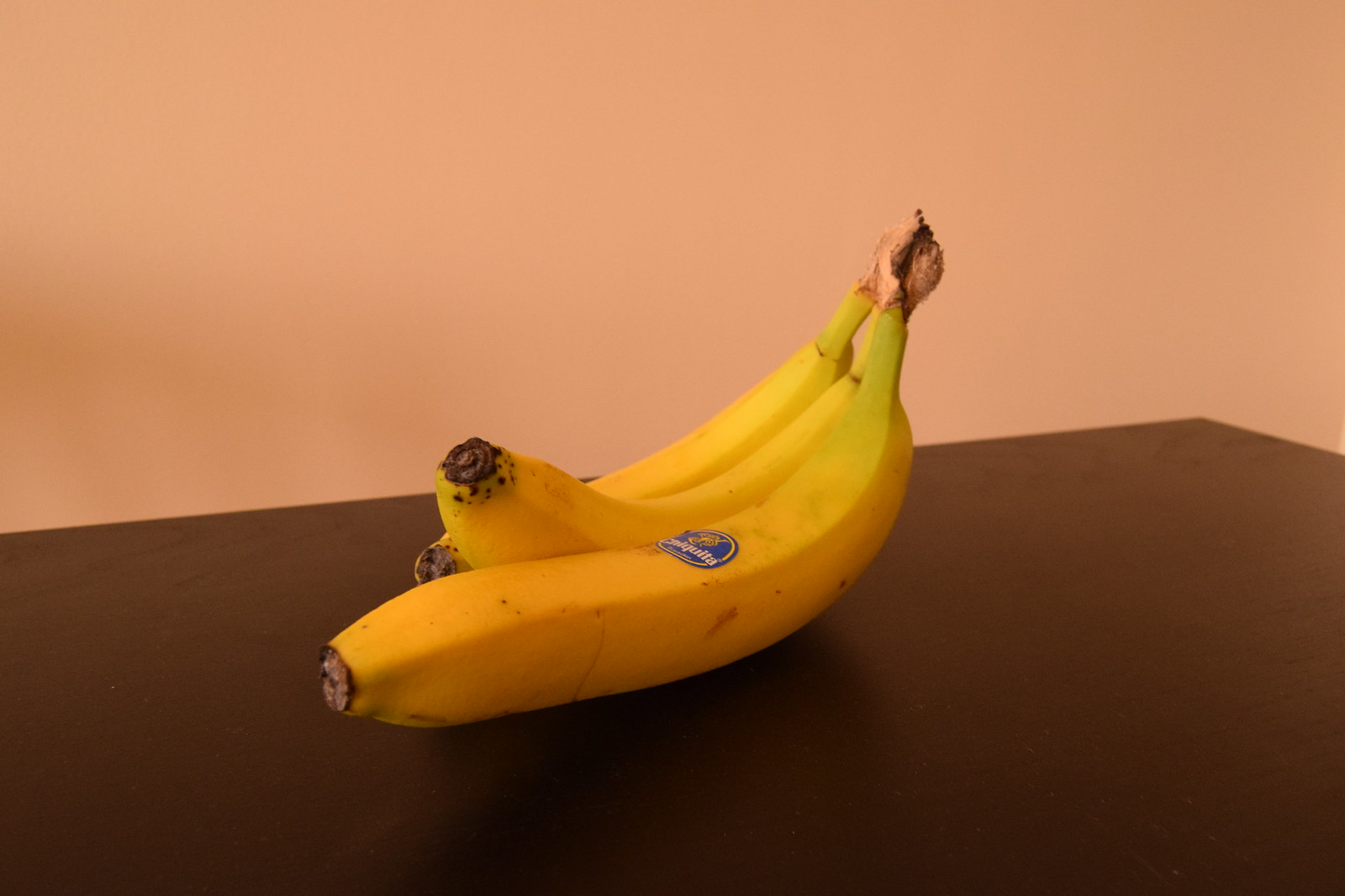This photograph showcases a trio of bananas resting on a dark brown wooden table. The bananas are still attached at the stem, which is notably brown at the tip. The stems exhibit a green hue, while the bananas themselves are perfectly ripe, adorned with a few small brown spots. The banana closest to the camera is the largest and features a blue sticker. Positioned in the middle, the second banana is about an inch shorter and curves upward. In the background, the smallest banana lies flat against the table. The backdrop of this scene is a lighter salmon-colored wall. The room appears to have moderate lighting, neither too dim nor overly bright, contributing to the photo's slightly blurry and unfocused quality.